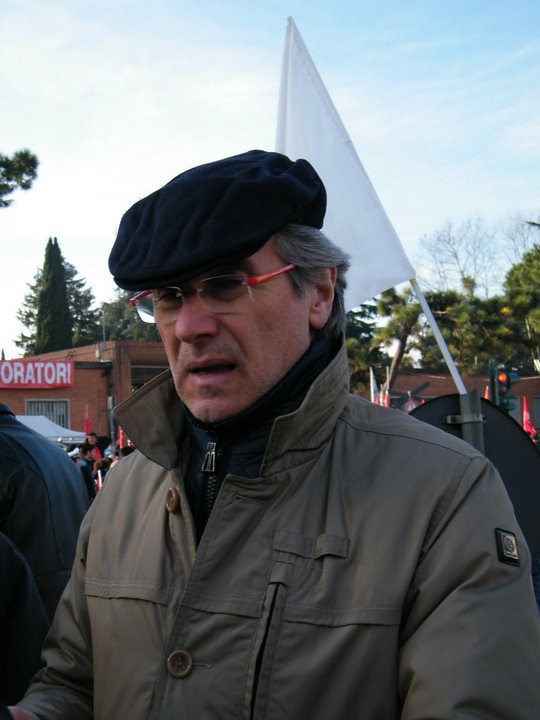In this image, a concerned-looking white man, appearing to be in his late 50s or early 60s, is the central figure. His silver-gray hair and five o'clock shadow are visible beneath a black beret. Red-rimmed glasses frame his worried eyes as he stares off to the side, beyond the frame. He is clad in multiple layers suitable for the cold weather: a brown windbreaker with buttons and a popped collar, over a black, zippered, high-neck sweater.

The background reveals a fairly crowded outdoor gathering or fair, with several people partially visible. A white triangular flag on a white pole, supported by a black holder, stands prominently behind the man's head. Farther back, the background features lush green trees and a mostly cloudy sky with streaks of blue. A red brick building with a partially visible red banner bearing white text that reads "ORATOR!" can be seen to the left. The scene suggests a chilly day amidst a communal event in a scenic, tree-lined area.